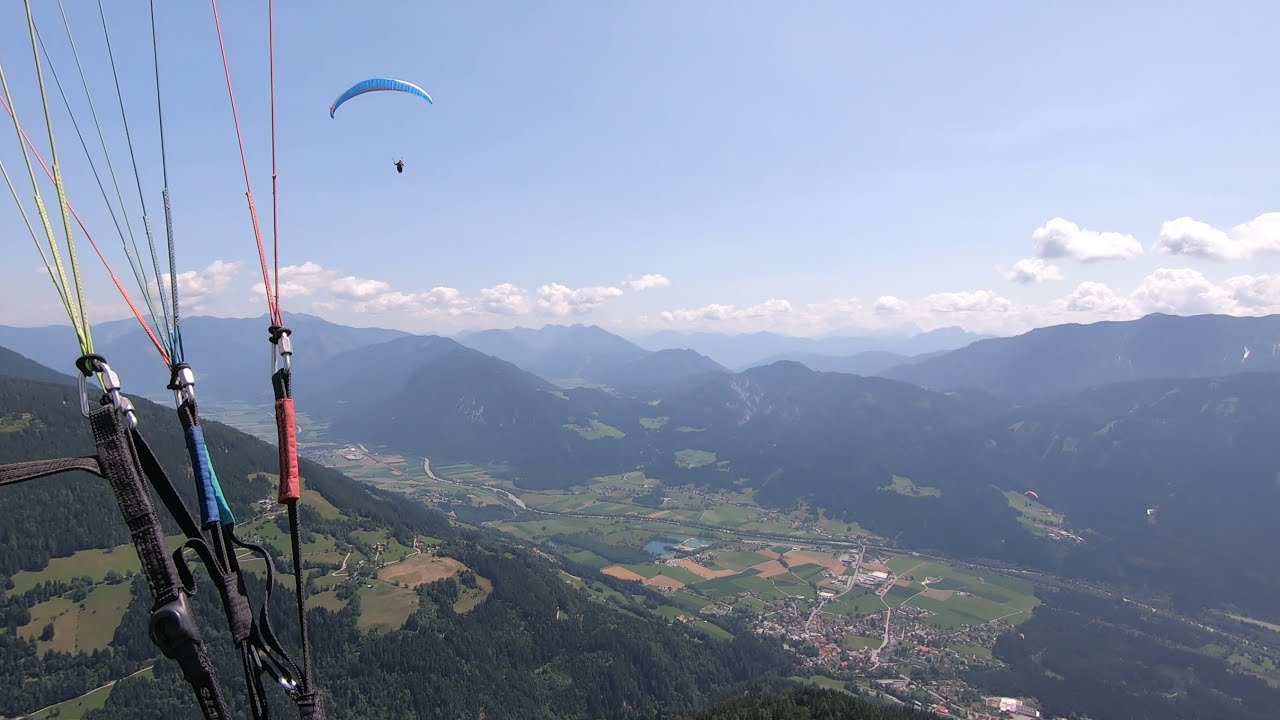This photograph appears to be taken from a high-altitude vantage point, likely from a GoPro or similar camera attached to a paraglider. The main focus is on two paragliders soaring in a pristine, expansive blue sky. One paraglider is prominently visible on the left side of the image, capturing the scene and giving us a view of the colorful parachute strings in red, black, and blue, leading up to the blue parasail. 

In the distance, another paraglider, with a light blue chute, floats gracefully amid the scattered white clouds. Beneath the paragliders, a stunning landscape unfolds, consisting of a valley enveloped by tall, densely treed mountains. The valley itself appears to contain a small town or city, identifiable by its buildings, suburban homes, roads, and perhaps even water sources. The time of day is suggested to be early evening, as inferred from the angle and quality of the sunlight. This serene and exhilarating bird's-eye view captures the exhilarating experience of paragliding over a picturesque and rugged terrain.